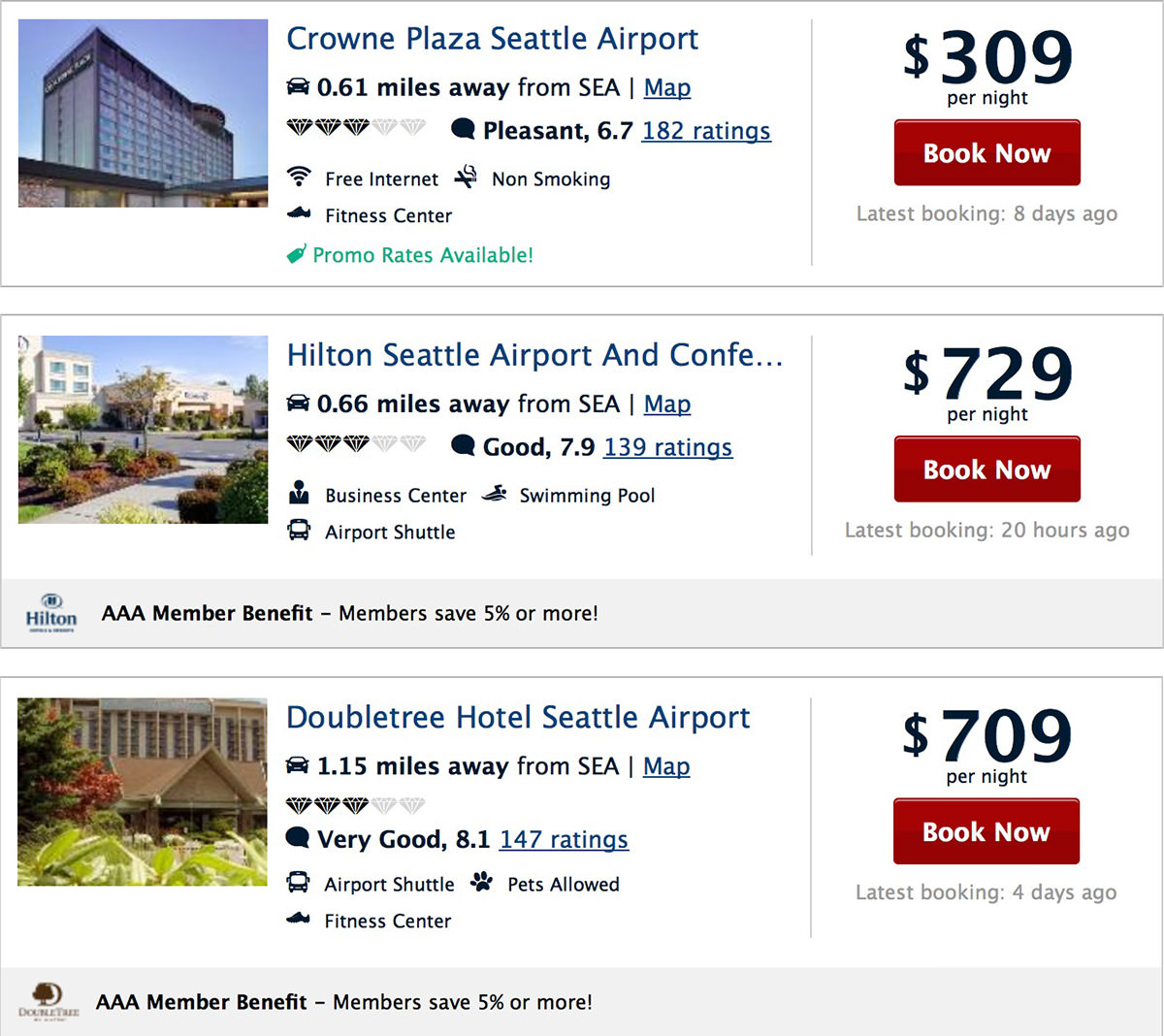This image depicts a hotel booking website interface showcasing three accommodation options near Seattle Airport (SEA). Each listing includes a picture of the respective hotel, brief information, and booking details.

1. **Crowne Plaza Seattle Airport**: The top listing features a large, gray-toned building identified as the Crowne Plaza, located 0.61 miles from SEA. The ratings show a score of 6.7, labeled as "Pleasant" based on 182 reviews. The nightly rate is displayed as $309, alongside a prominent "Book Now" button.

2. **Hilton Seattle Airport & Conference Center**: The middle option displays an image of a slightly smaller hotel with surrounding trees. This Hilton property is situated 0.66 miles from SEA and carries a rating of 7.9, classified as "Good." The nightly cost for this hotel stands at $729, positioned above the "Book Now" button.

3. **Doubletree Hotel Seattle Airport**: The final hotel listing shows a larger building with a distinctive brown roof and a pointed awning. Named the Doubletree Hotel, it is located 1.15 miles from SEA. With a rating of 8.1, categorized as "Very Good," this accommodation is priced at $709 per night, with a book now option prominently available.

Each listing includes pertinent details that aid in making an informed booking decision.